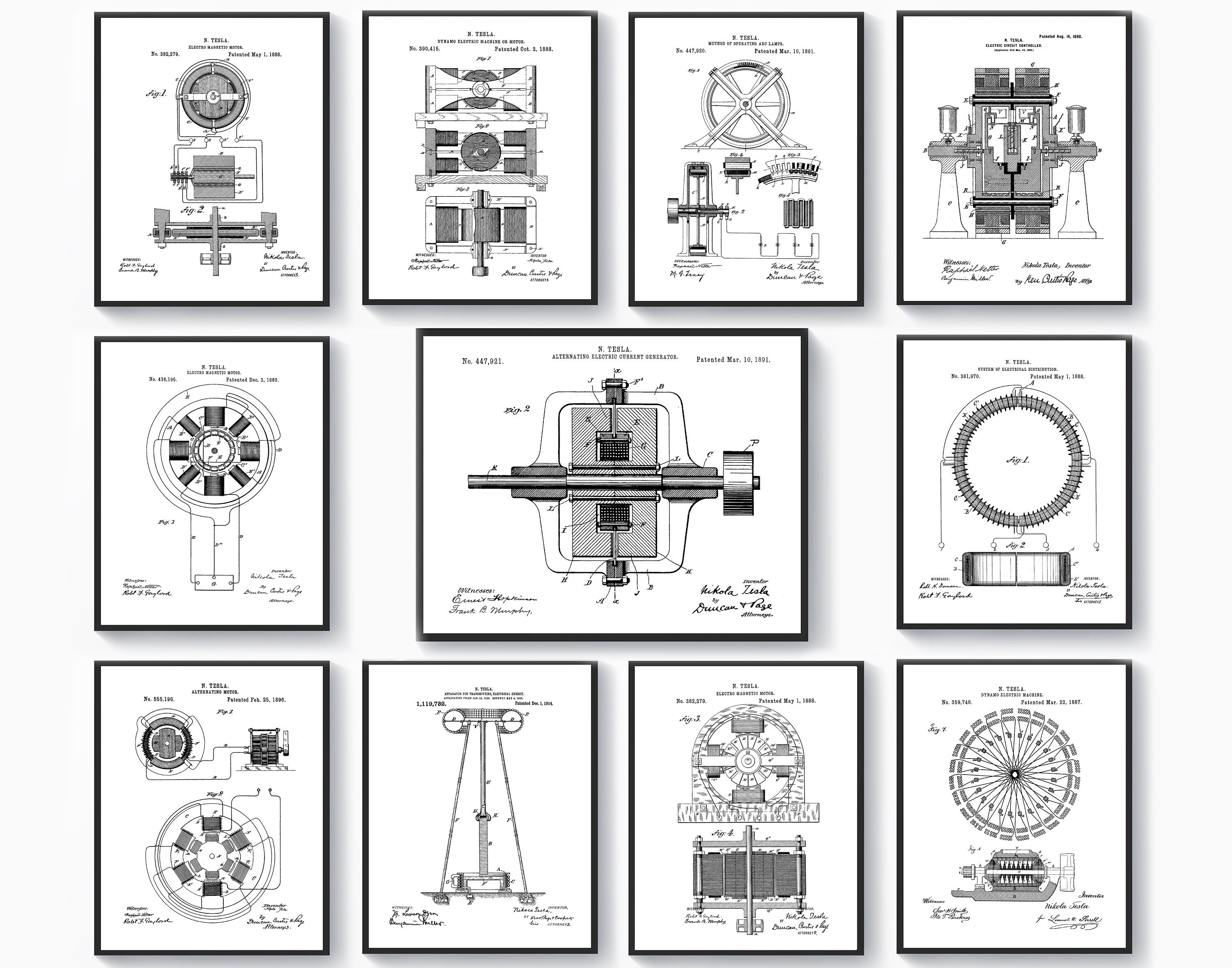The image depicts a series of 11 detailed black-and-white diagrams of various pulley systems and machinery components, organized in a grid pattern on a white background with black borders around each drawing. The layout consists of three rows: the top and bottom rows each contain four equally-sized pictures, while the middle row features a smaller picture on the left, a significantly larger central image, and another smaller picture on the right. Each diagram appears to illustrate different parts and mechanisms of a complex machine, with some drawings resembling historical sketches in the style of Da Vinci's notes. The details include gears, rods, and other mechanical elements, which collectively seem to showcase the inner workings and assembly of the machinery. There is also a subtle shadow behind each frame, suggesting that the photo might have been taken of a display on someone's wall.